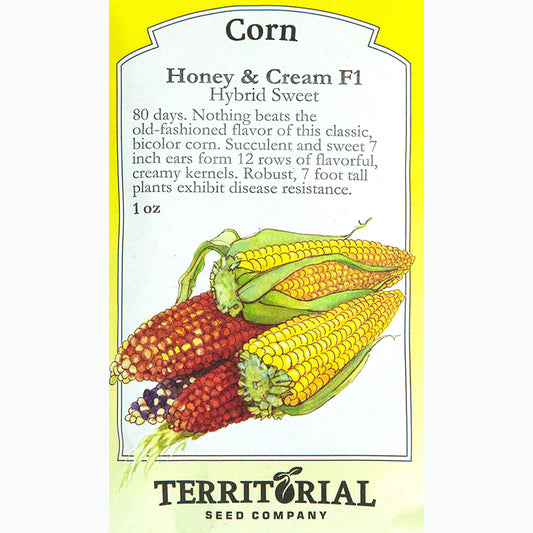This image depicts a computer-generated representation of a packet for corn seeds, specifically the "Honey and Cream F1 Hybrid Sweet" variety. The packet has "Corn - Black" prominently displayed at the top. Below this title, detailed descriptions are provided: 

- The seeds are expected to produce corn in approximately 80 days.
- The corn variety boasts an old-fashioned flavor, offering classic bicolor ears that are succulent and sweet.
- The ears measure about seven inches and contain 12 rows of flavorful, creamy kernels.
- The robust plants grow to about seven feet tall and exhibit disease resistance.
- The packet size is indicated as one ounce.

Visually, the packet features five illustrated ears of corn with distinct colors: two yellow, two reddish, and one purple, some with portions of their husks still attached. The bottom of the packet displays the "Territorial Seed Company" branding. Surrounding the design is a yellow border, enhancing the appearance of an actual seed packet.